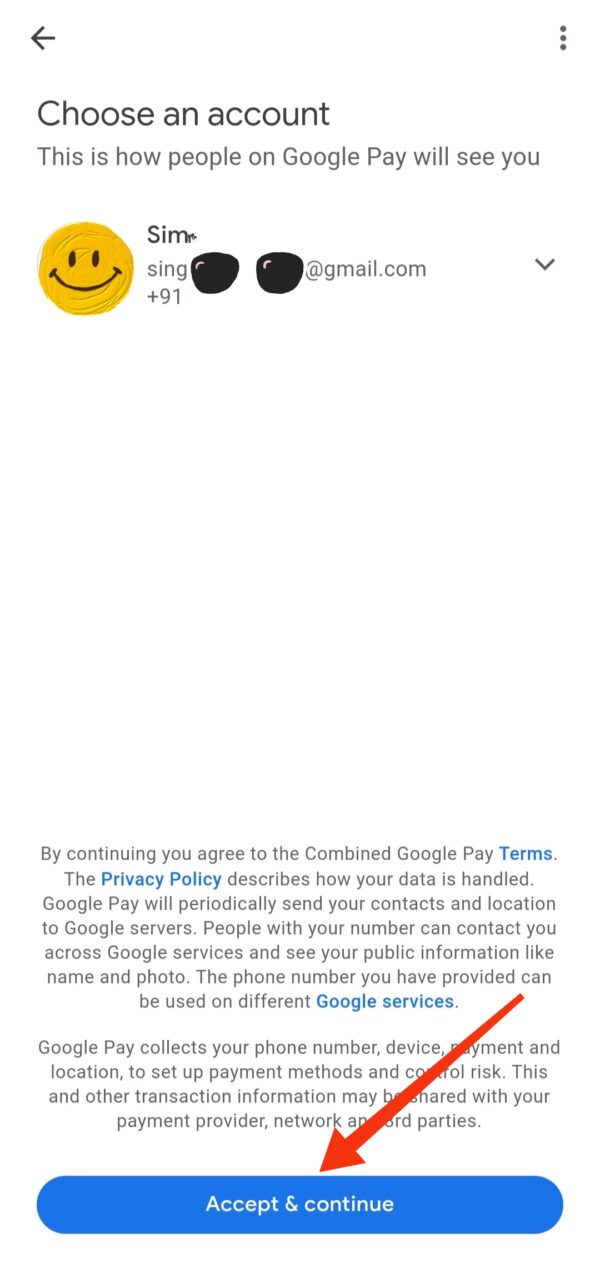The image displays a Google Pay setup page, prompting the user to choose an account. The screen features a single account option with a profile picture of a stylized black smiley face against a yellow background, giving it a painted and textured appearance. The account is labeled "sim," with part of the email address visible as "sing****@gmail.com;" the portion after "sing" is obscured by a graphic resembling sunglass lenses for a playful touch. The majority of the screen is filled with legal text explaining the terms and privacy policy, detailing how data is managed and associated with the Google Pay service. At the bottom, there's a prominent blue "Accept & Continue" button, highlighted by an edited red arrow directing attention to it. The overall look and function of Google Pay are likened to Apple Pay for iPhone users, indicating similar functionality across the platforms.